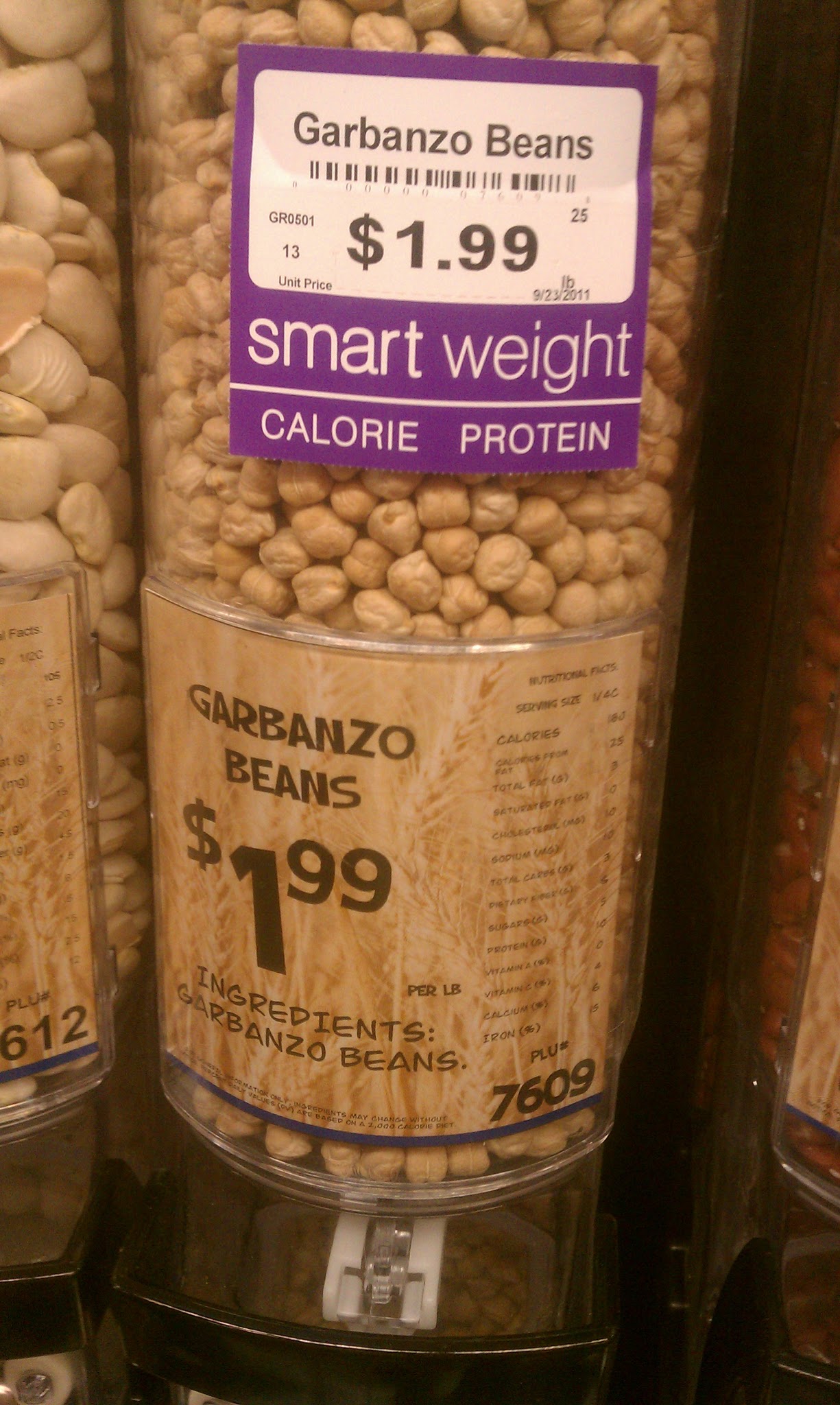This photograph captures a bulk section of a grocery store, prominently featuring a cylindrical, tall plastic container filled to the brim with dried garbanzo beans. The container is part of a larger display with similar dispensers for various beans, visible on both sides, potentially containing larger beans and possibly red beans, although these are less discernible.

The garbanzo bean container is well-labeled: a sticker at the top marks it clearly with "Garbanzo Beans" in bold letters. Below this, a price tag indicates a cost of $1.99 per pound. Additionally, the label includes essential nutritional information, although it's too small and blurry to read in detail, except for the ingredients listed as "Garbanzo Beans." The PLU number 7609 is also visible on the label.

A purple, black, and white sale price tag outside the container features the text "SmartWeight" along with keywords "calorie" and "protein," and a barcode. The barcode displays "612," enhancing the detailed itemization. The overall design of the label incorporates a wheat motif in beige and brown tones, adding a subtle touch to the practical display.

Finally, a dispensing mechanism is situated at the bottom of the container, allowing customers to release the beans as needed. This image meticulously presents the simplicity and functionality of bulk grocery shopping.